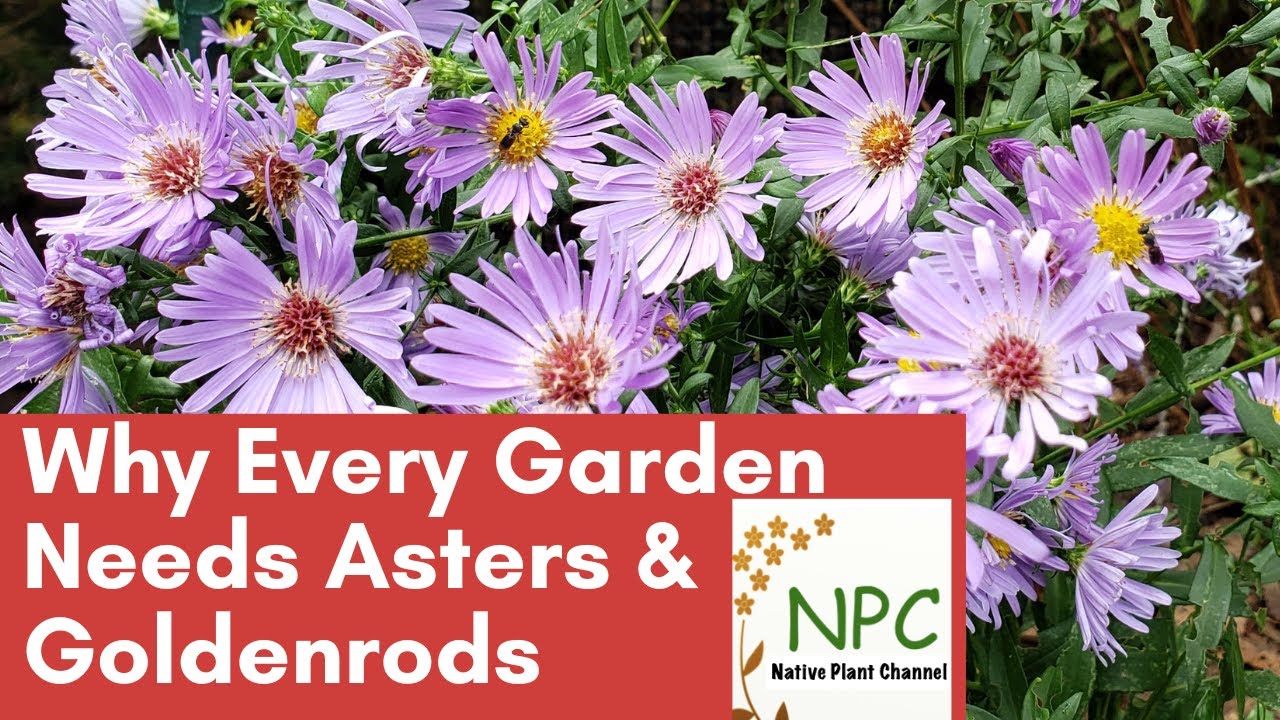This image seems to be a promotional poster or cover for an informational booklet or advertisement. It features a vibrant, color photograph of beautiful pinkish-purple asters with some having golden yellow centers and others with rich purple centers. The background is filled with lush green foliage and several bugs diligently working on the multiple blooms and buds, enhancing the fresh and sunny ambiance of the scene. 

Dominating the lower right corner and extending two-thirds across the image is a striking pink or red block of color. This block contains text in bold white letters that reads, "Why Every Garden Needs Asters and Goldenrods," suggesting that these are the names of the featured flowers. 

In the bottom right corner of this color block is the logo for the Native Plant Channel (NPC). The acronym "NPC" is prominently displayed in green letters, with "Native Plant Channel" written beneath in black block letters. Adjacent to the NPC logo is a graphic element of a stem with golden five-tipped stars emerging from it, resembling either flowers or decorative stars.

Overall, the poster conveys not only the beauty of these garden plants but also the educational and promotional messaging from the Native Plant Channel.